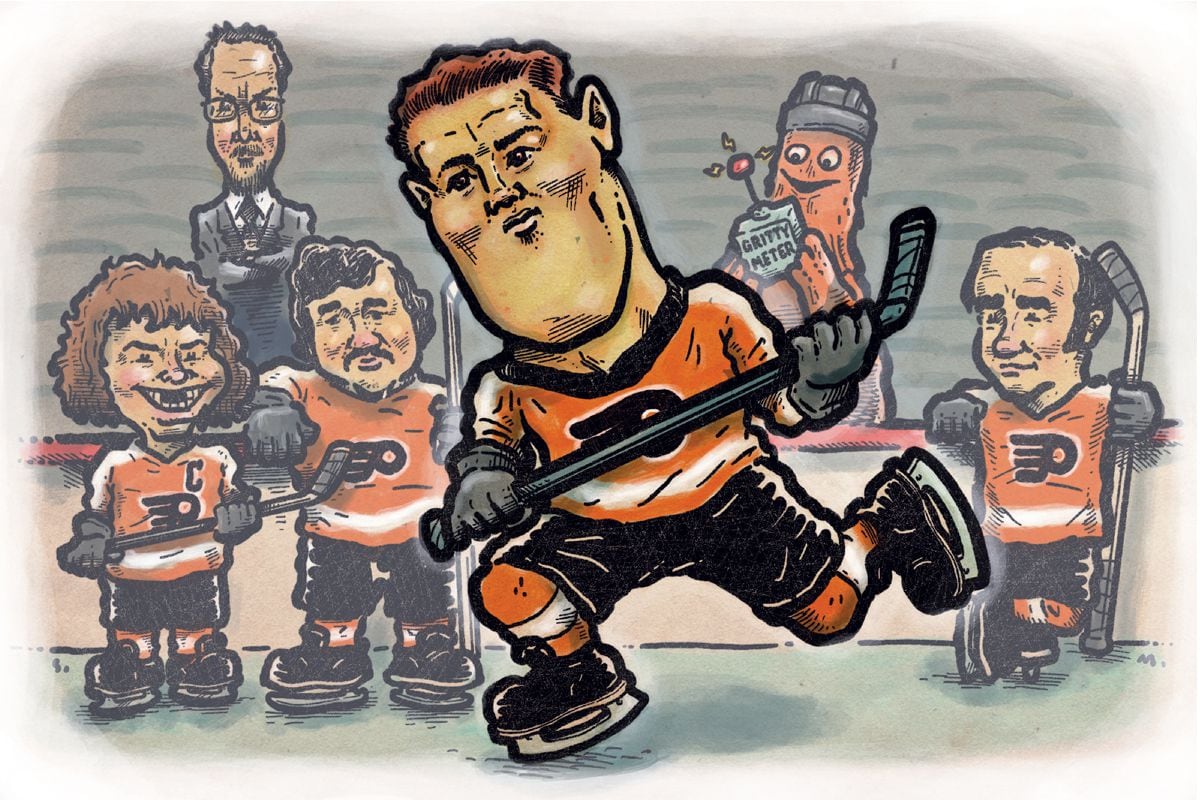This hand-drawn caricature-style cartoon depicts members of the Philadelphia Flyers ice hockey team. The drawing is set in landscape mode and prominently features the team's mascot, a big, fluffy orange figure, known as Gritty, who is situated in the background on the right-hand side. Gritty is wearing a hockey helmet and holding up a small box labeled "gritty meter." To the left of Gritty stands a tall, slender man with glasses who appears quite displeased as he looks out over the ice.

The foreground of the illustration showcases four hockey players, all wearing the iconic orange jerseys of the Philadelphia Flyers, complete with black collars, white stripes, black shorts, and orange socks with white stripes. They have black ice skates with silver blades. The players are in exaggerated caricature style, with unusually large heads. The leftmost player is missing his front teeth; the player next to him sports a mustache, while another player leans casually against the side of the arena. The most prominent figure, dominating the front of the cartoon, features an extremely large chin and is actively skating as part of the game.

The ice beneath them is depicted in shades of light and dark green, adding a whimsical touch to the scene. The players' movements are suggested through stylized lines, imitating wind to emphasize their speed and dynamism. The scene captures both the intensity and the playful spirit of the team and their mascot.